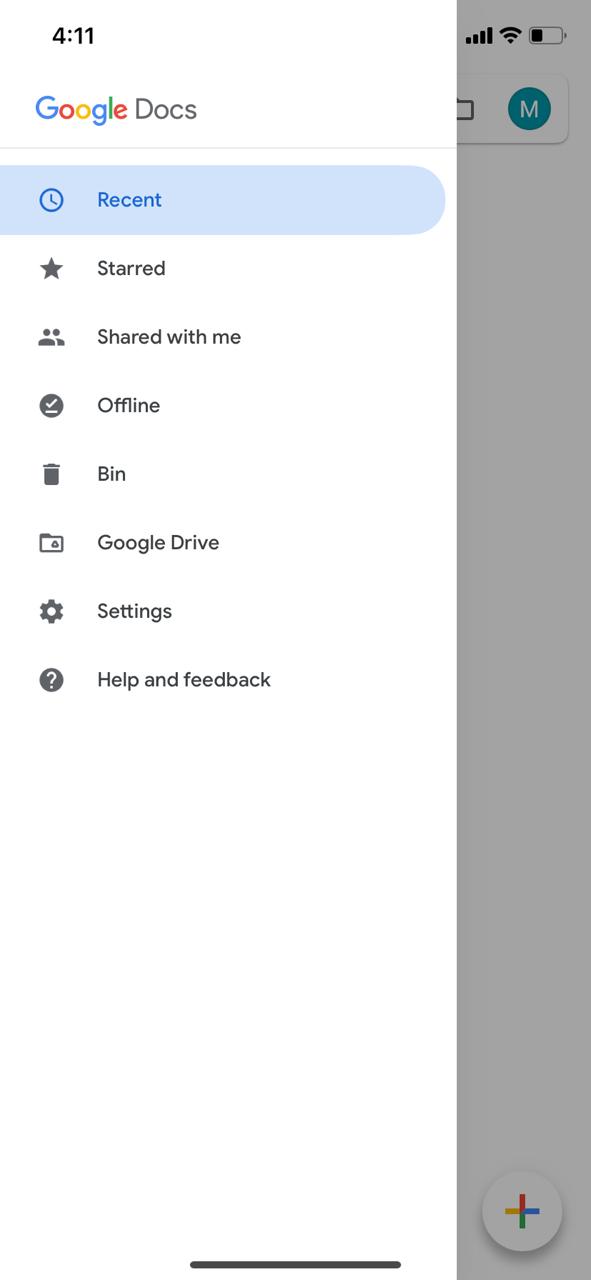The image captures a mobile screen displaying the Google Docs application. At first glance, it's clear that this is not a Google Search but the Google Docs interface. The screen is mostly in black and white, except for the colorful Google logo in blue, red, yellow, and green, and some highlighted elements in blue. 

The text on the screen mentions "Recent," "Start," "Shared with Me," "Offline," "Bin," "Google Drive Settings," and "Help and Feedback," with "Recent" being selected. There is a slight darkness on the right-hand side of the screen, indicating that certain options are being highlighted while the darker areas are not selected. 

The time displayed at the top left corner is 4:11, and the right side shows status indicators for cellular bars, more bars, battery life, and the letter "M," possibly denoting the user's name, which could be Michael. The design is simplistic and minimalistic, emphasizing functionality. 

At the bottom center of the screen, a distinct line demarcates the area, suggesting that this is a mobile device. The overall aesthetic of the image is clean and focused on essential elements for easy navigation and usability.